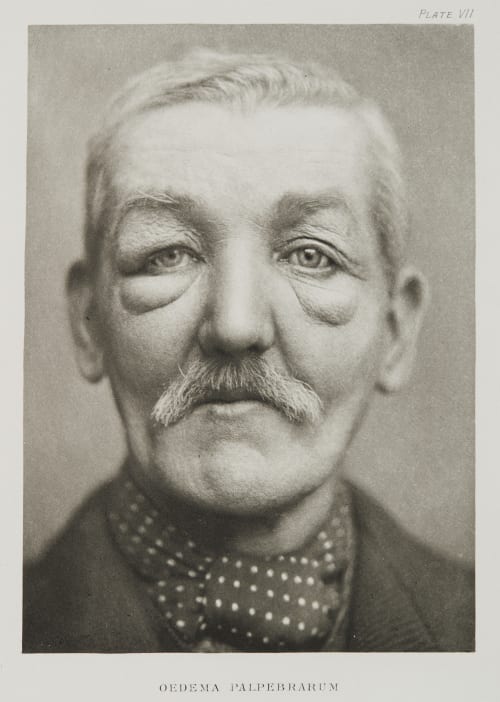This black-and-white photograph, measuring approximately 6 inches high by 4 inches wide, features an older man gazing straight at the camera. The image is set within a thin gray border, with the inscription "Plate B-I-I" at the top right corner and "O-E-D-E-M-A P-A-L-P-E-B-R-A-R-U-M" at the bottom center in light gray print. The man has a long, narrow face with short white hair and a white mustache. His eyes are notably heavy-lidded with pronounced bags underneath, giving him a weary appearance. He is dressed in what appears to be a dark-colored sweater, accompanied by a dark tie adorned with white polka dots. The backdrop behind him is a light gray shade, enhancing the contrast with the detailed features of his face and attire.